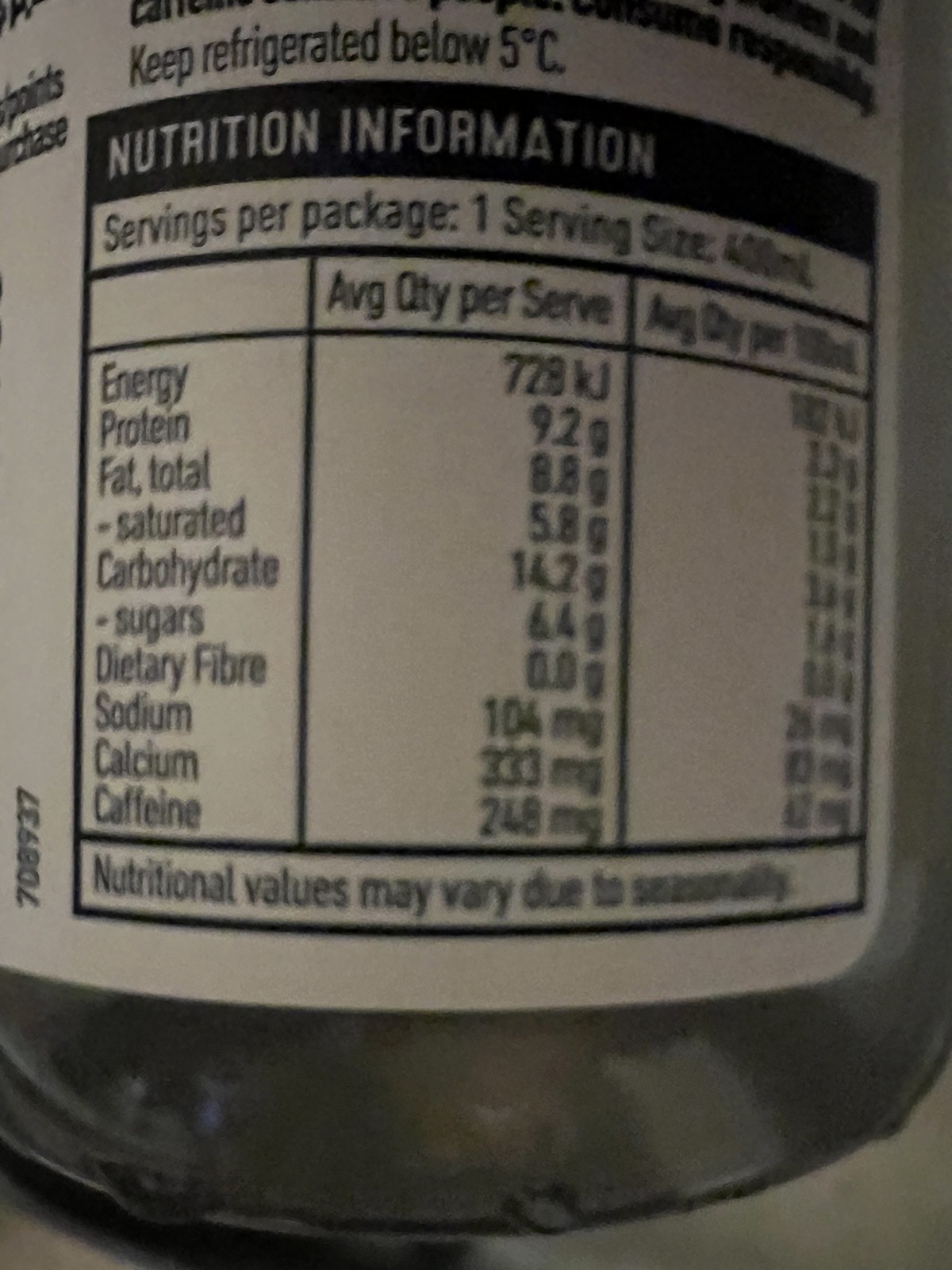This image captures the nutrition information label of an unidentified refrigerated product. Displayed prominently in a clear and structured square box, the label provides essential details for consumers. At the top, it notes a storage instruction: "Keep refrigerated below 5°C." Below this, the nutritional information is meticulously categorized, listing key components such as energy, protein, total fat, saturated fat, carbohydrate, sugars, dietary fiber, sodium, calcium, and caffeine. The product offers one serving per package, with a serving size of 400 milliliters. Notably, it includes caffeine, suggesting it may be a beverage or a caffeinated food product. The use of the spelling "fibre" and the metric units strongly indicates that the product is intended for the English market outside of the USA.